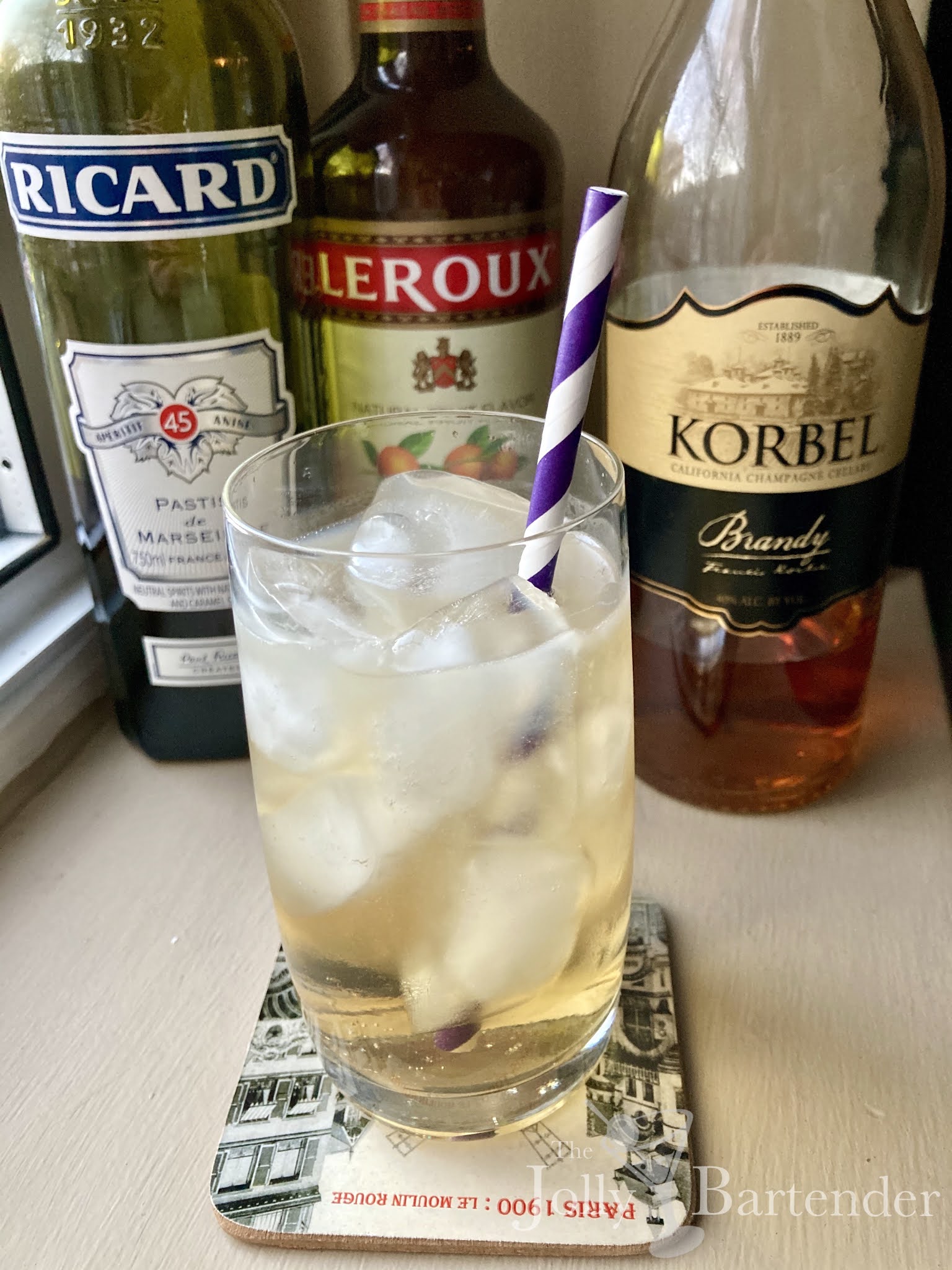This detailed indoor tabletop photograph captures a well-curated selection of liquor bottles and a prepared drink. Central to the image is a clear glass filled with ice and a slightly yellow-tinged liquid. Sticking out of the drink is a distinctive purple and white striped paper straw. This glass rests on a paper coaster that features the text "Paris 1900 Les Moulins Rouge." Behind the drink, three bottles are arranged: a green bottle with white and blue labels prominently displaying "Ricard 45 Aperitif Anise," a dark-colored bottle labeled "La Rue," and a nearly empty clear bottle with black and beige labeling that reads "Corbel California Champagne Brandy." The photo is subtly branded with a watermark in the bottom right corner, showcasing a martini glass icon alongside the text "The Jolly Bartender" in white print.